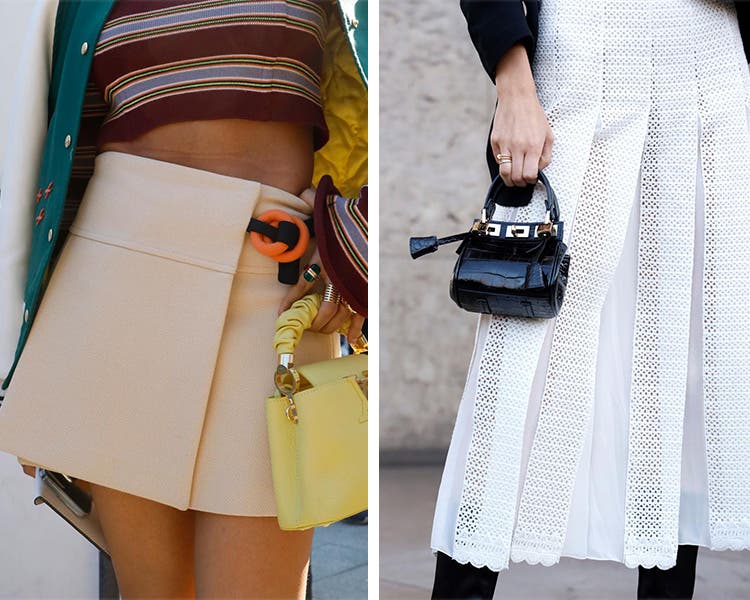This side-by-side product shot features detailed images of two women modeling different handbags. The left image captures a very thin, bronze-skinned woman dressed in a cream-colored miniskirt accentuated by a black tie and orange rings around the waist. She pairs the skirt with a cropped, brown long-sleeve shirt, and a green and white letterman's jacket with three gold buttons. Her right hand holds a small yellow handbag with a ribbon handle and gold accents, and she sports stylish jewelry on her fingers. The right image portrays a woman in a long, white skirt with a mesh overlay and black boots. She is holding a very small micro handbag made of black patent leather with gold accents. Her outfit is completed with a white sundress, emphasizing a fashionable, cohesive look.